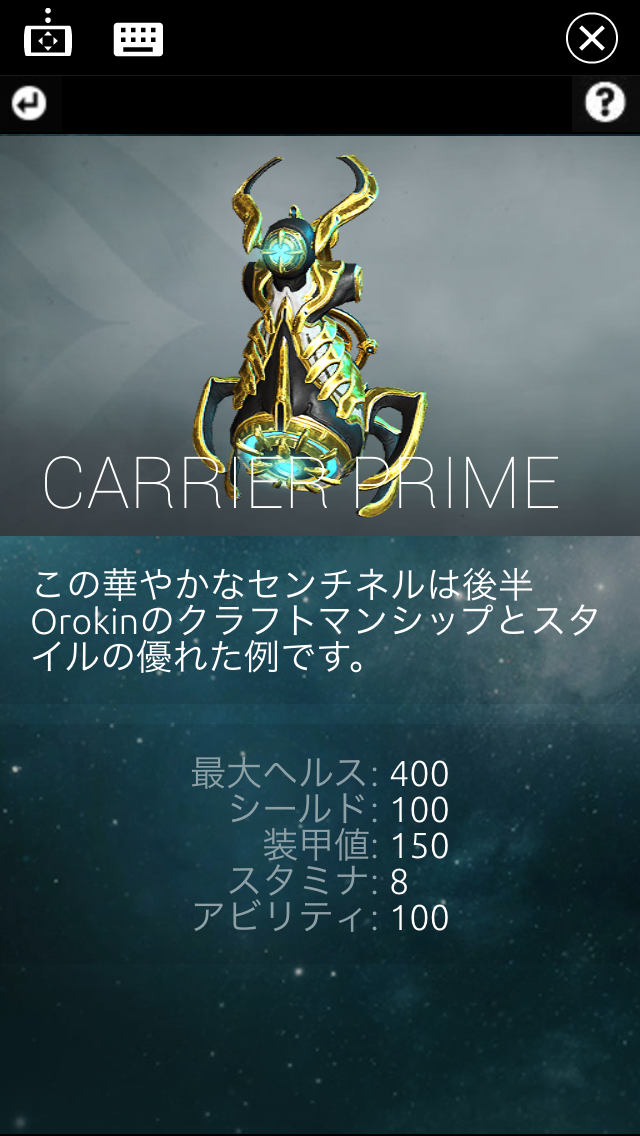The image appears to be a screenshot taken from a mobile device, likely while playing a game, as suggested by its rectangular shape. The long sides of the image are on the left and right-hand sides, while the short sides are at the top and bottom. The image features a black rectangular border with various icons and details. In the top right corner, there's an 'X' button encircled, which seems to be for closing the screen. Just below it is a question mark icon, indicating help or information. On the left side, there's a small icon resembling a keyboard and an arrow pointing left, likely a back arrow to exit the screen.

At the center of the image, the main focus is on a vibrant, metallic object named "Carrier Prime." This object has an insect-like appearance, resembling a beetle or perhaps a scorpion, with a body that is gold in color and blue light emanating from it. It also features golden tentacles or antennae protruding from its head, adding to its ornate look. The name "Carrier Prime" is prominently displayed below this object. Surrounding it, there is Japanese text along with numbers arranged from top to bottom, which include 400, 100, 150, 8, and 100, likely indicating some form of stats for the creature or object. Additionally, the name "Orokin" accompanies the image, adding further context to its ornate design and possibly its origin within the game.